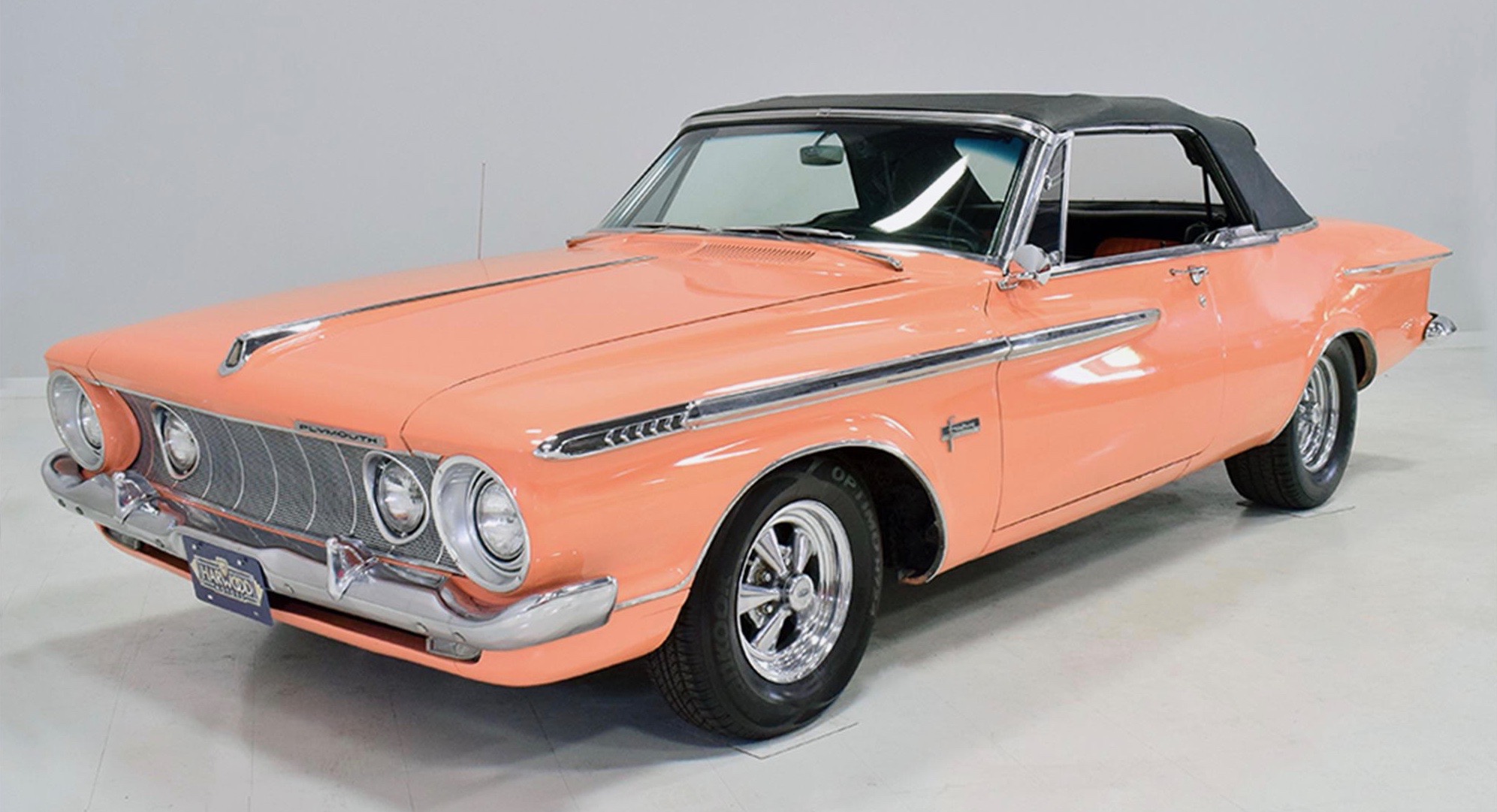This is a detailed photograph featuring a classic American muscle car, specifically identified as a Plymouth by the emblem on its hood. The car boasts a distinguished peachy, light pastel orange paint job that gleams under the light, reflecting beautifully off its polished surface. The convertible's black top is currently closed, and the car is positioned diagonally, showcasing its sleek profile. The vehicle is parked in what appears to be a pristine showroom or garage with an impeccably clean white floor and walls, adding to its presentation. Notably vintage, the car is reminiscent of models from the 1960s, with signature chrome detailing, including shiny silver bumpers and rims, as well as black tires. The front end features a distinctive roundish grille housing four round headlights, further enhancing its classic look. The overall pristine condition and the meticulous detailing of the black and chrome interior highlight the car's well-preserved state, making it a stunning example of automotive history.